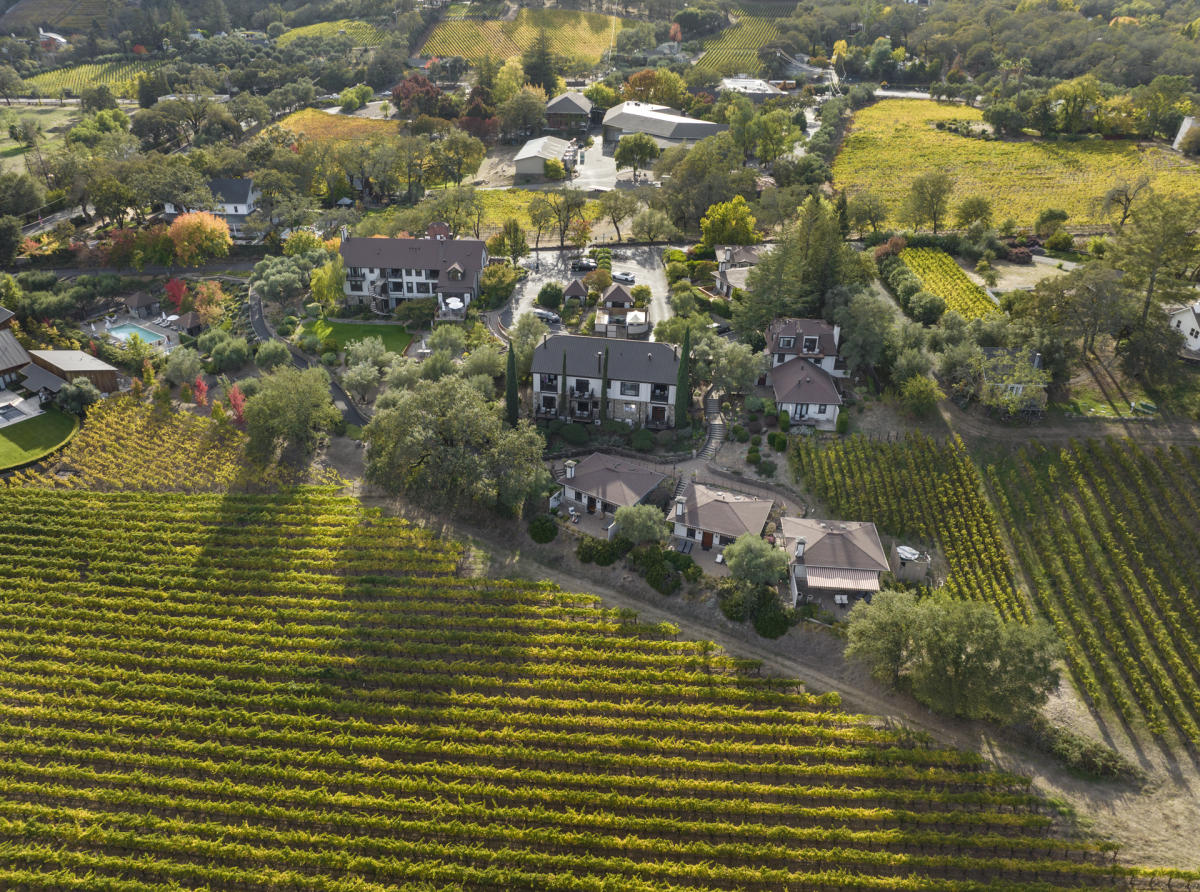An aerial photograph of a vibrant farmland captures a detailed landscape featuring numerous fields, buildings, and roads. In the lower left portion of the image, dozens of rows of green crops are neatly aligned, stretching horizontally. The right side of the photo showcases additional rows of the same crop, along with several smaller plots in the upper right corner. The middle section reveals two large, white houses with gray roofs, surrounded by five smaller single-story homes, forming a cluster of residences. One of the main houses is distinguished by three Italian cypress trees adorning its entryway. A diagonal road begins at the lower left side, branching into a fork with pathways extending from the same location. Additional scattered homes dot the hillside, amidst a scattering of trees and gentle hills. Adding to the idyllic setting, a swimming pool is situated in the upper mid-left section of the image, enhancing the inviting atmosphere of this bustling farming community.